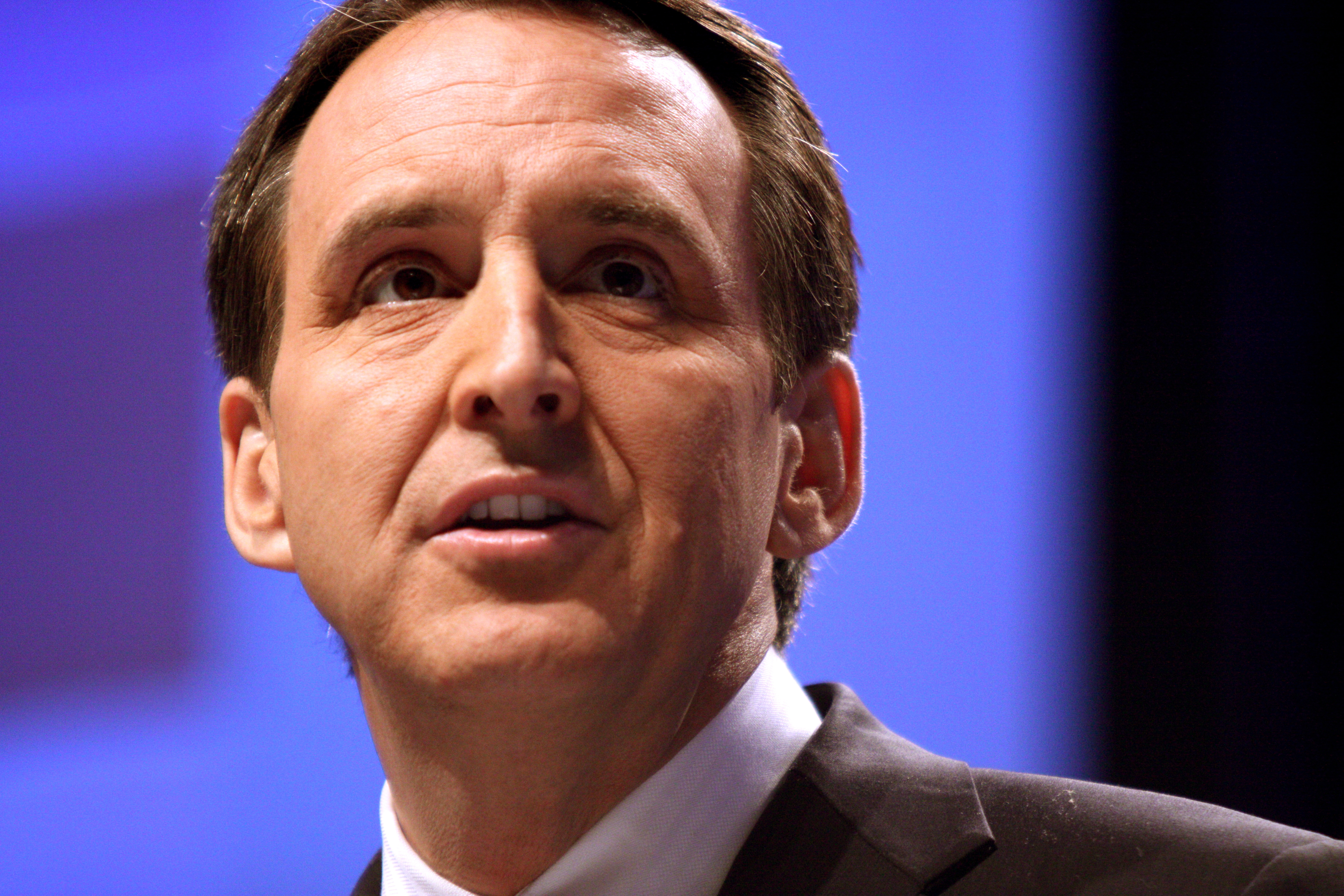This is a highly zoomed-in photograph of a man, framed from his upper shoulders to just below the top of his head, which is slightly cut off by the edge of the image. The man, who appears to be in his 40s or 50s, has short brown hair combed to the side and brown eyes that are directed upwards. He is wearing a dark gray business coat over a collared white button-up shirt. His mouth is partially open, revealing his upper teeth, as if he is mid-speech. Behind him, there is a large, blurry projection screen with a noticeable red rectangle in the middle, and to the right of the screen, the background is pitch black.